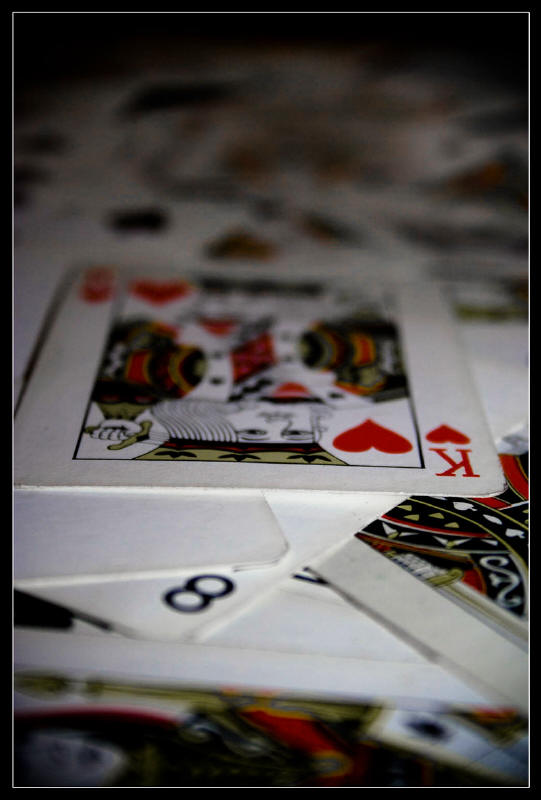A vertically oriented, color-altered photograph, possibly edited using Photoshop, surrounded by a black border. Central to the image is a sharply focused King of Hearts, with his face and the heart symbols in moderate focus. The upper part of the King of Hearts card gradually blurs into an abstract blend of colors. The side edges of the card are visible, but the back edge seamlessly blends into the background, adding to the artistic effect. In the foreground, an Eight of an indeterminate suit (either Clubs or Spades) lays atop other cards, obscuring its suit symbols. Below the Eight, another face card (a King, Queen, or Jack) is partially visible, creating a layered, dynamic design as if the cards were tossed carelessly. The bottom border of the image reveals a sliver of another card, very blurred, adding to the depth and complexity. The palette includes shades of red, light olive green, black, white, and a yellowish-green, contributing to the image's surreal and artistic aesthetic.